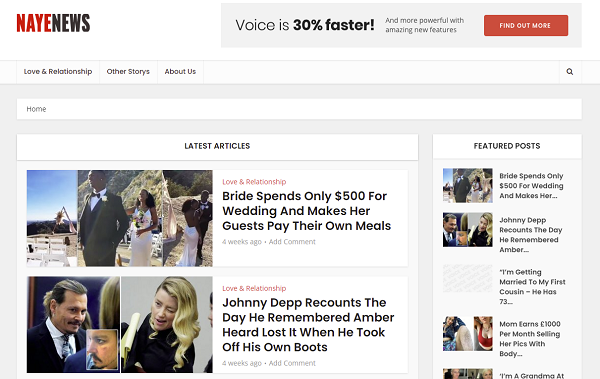This image presents a webpage from the NAYE News website, set against a white background. Prominently displayed in the upper left corner is the site's title: "NAYE" is in red, bold text, followed by "NEWS" in black, bold text. In the upper right, there is a light gray banner with black text that highlights, "Voice is 30% faster," with the "30% faster" part emphasized in bold. Adjacent to this in smaller gray text is the phrase, "and more powerful with amazing new features." A red button to the right reads "Find out more" in white text.

Below the header, there are three navigation buttons on the lower left: "Love and Relationship," "Other Stories," and "About Us." The featured article on the left is titled, "Bride spends only $500 for wedding and makes her guests pay for their own meals," displayed in bold black text. To the left side of this article is an outdoor photograph depicting a bride in a white dress with the groom standing in front of her.